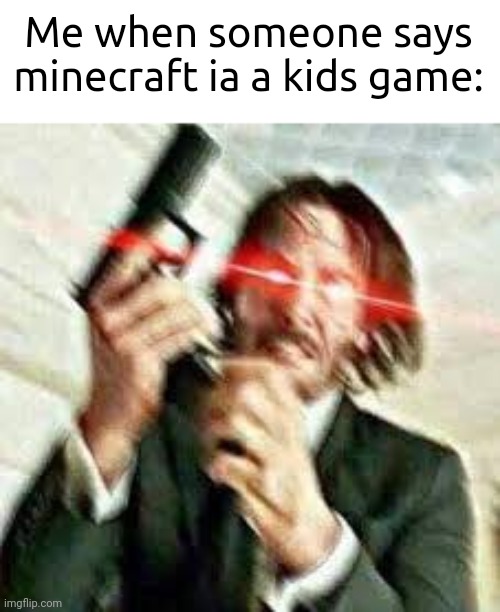A dynamic and intense image captures a scene from one of the John Wick movies, featuring the titular character, John Wick, in the midst of a high-adrenaline moment. Large text at the top of the image boldly proclaims, "Me when someone says Minecraft is a kid's game." In this visually striking depiction, John Wick's face is contorted into a furious expression, teeth gritted, and his eyes emit an ominous red glow with laser beams shooting outwards. He is in the act of reloading his gun with a fresh magazine, emphasizing his enraged and combative state. This powerful illustration serves as a commentary on the widespread appeal of Minecraft, highlighting that it is a game enjoyed by people of all ages and demonstrating that it transcends the label of being merely a child's game.